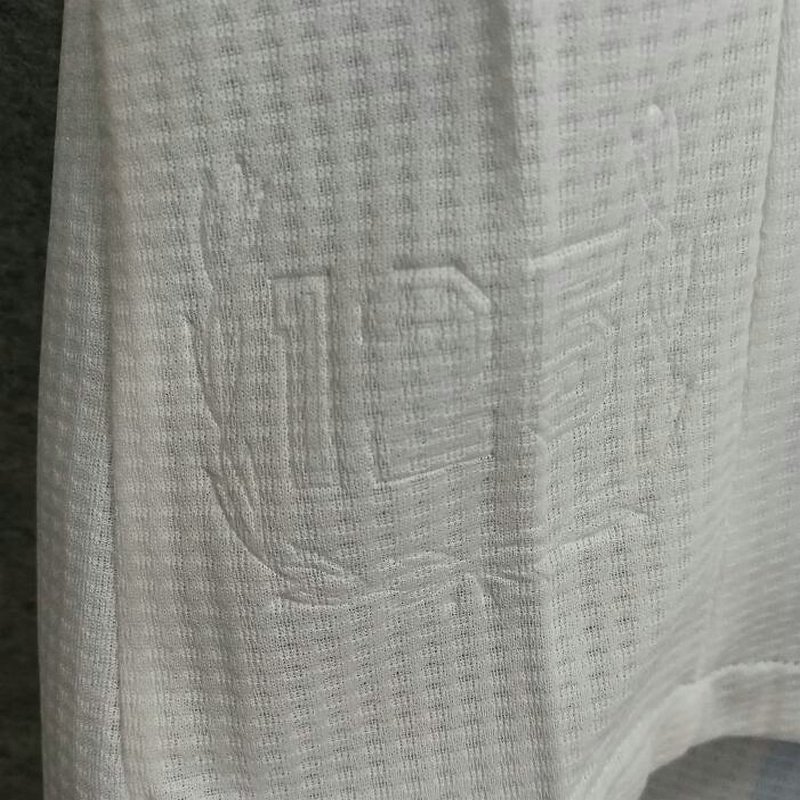The image features a white drapery, potentially a blanket or window curtain, characterized by a semi-transparent, checkered weave pattern. The drapery is adorned with intricate embroidery resembling twisting vines that extend from the center towards the left, right, and upwards. Within the embroidery, the text "125" is visible, likely indicating a brand logo. The drapery is suspended above a grey carpet and is positioned against what appears to be a grey wall. There is a noticeable center crease in the fabric, suggesting it could benefit from ironing.